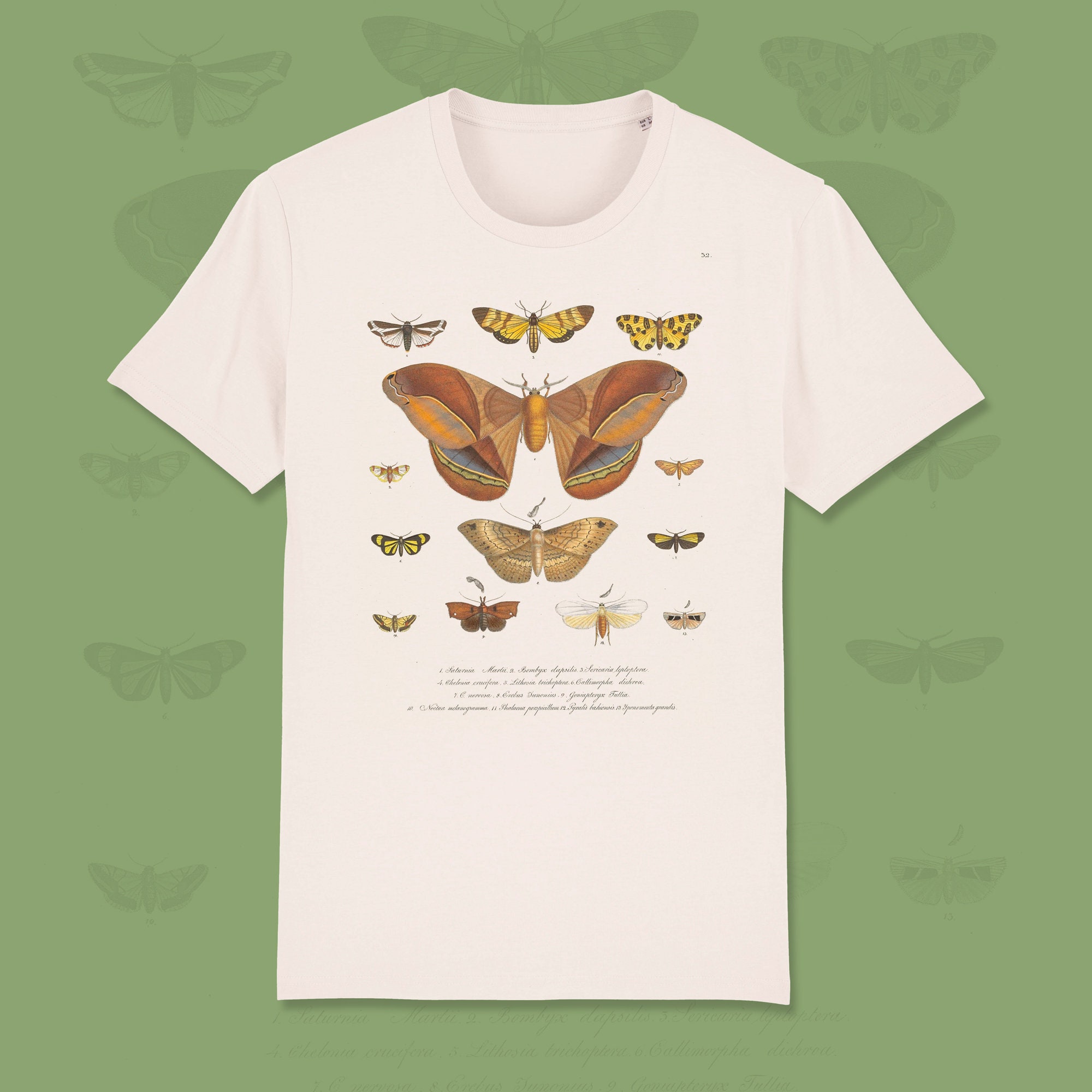This photograph features an off-white, cream-colored crew neck t-shirt laid on a sage green background adorned with silhouettes of moths in various shapes. The t-shirt, which has short sleeves, is decorated with a plethora of moth images, varying in size and color patterns. Dominating the upper center of the shirt is a large, detailed moth with brown, tan, and gray hues, its broad wings distinctly visible. Surrounding it are multiple smaller moths, including a notably large one positioned at the bottom center. These moths showcase a range of colors from yellows and browns to beiges, often with intricate spotting and array patterns. Below the ensemble of moths, there are three lines of script text in black, although the text is too small to be legible.